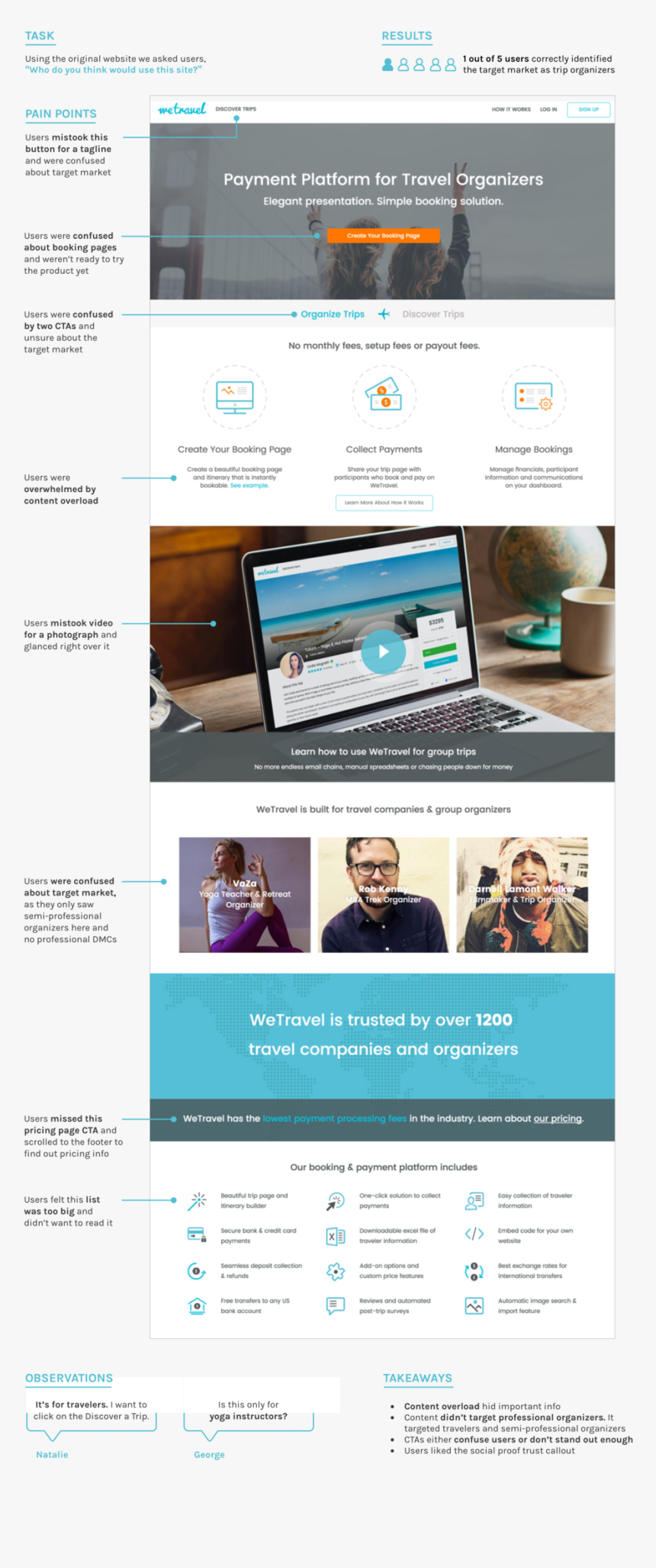The image appears to be a partial screenshot of a webpage, possibly viewed on a cell phone or computer. The screenshot is vertically oriented and features a white background with black text. At the top, there's a section labeled "Task" in blue, with "Results" to its right.

Under the "Task" heading, the text reads: "Using the original website, we asked users: Who do you think would use this site?" Below this, an illustration shows one out of five silhouetted figures highlighted, accompanied by the text: "One out of five users correctly identified the target market as trip organizers."

Beneath this, a large gray box contains text that describes the site's offerings: "Payment platform for travel organizers, elegant presentation, simple booking solution." Adjacent to this text is an orange clickable bar.

Further down, the screenshot includes another rectangular area featuring an image of a computer screen displaying a beach scene. In the center of this image is a blue circle with a play button (triangle) icon.

The screenshot continues with a section showcasing three photographs: one of a woman exercising, another of a man with glasses and a purple shirt smiling at the camera, and a third image of a black man wearing a hat and making a playful fish-lips gesture.

At the bottom, there's a blue box stating: "WeTravel is trusted by over 1,200 travel companies and organizers."

Overall, the image appears to be detailing a webpage for WeTravel, a company offering travel organization solutions.